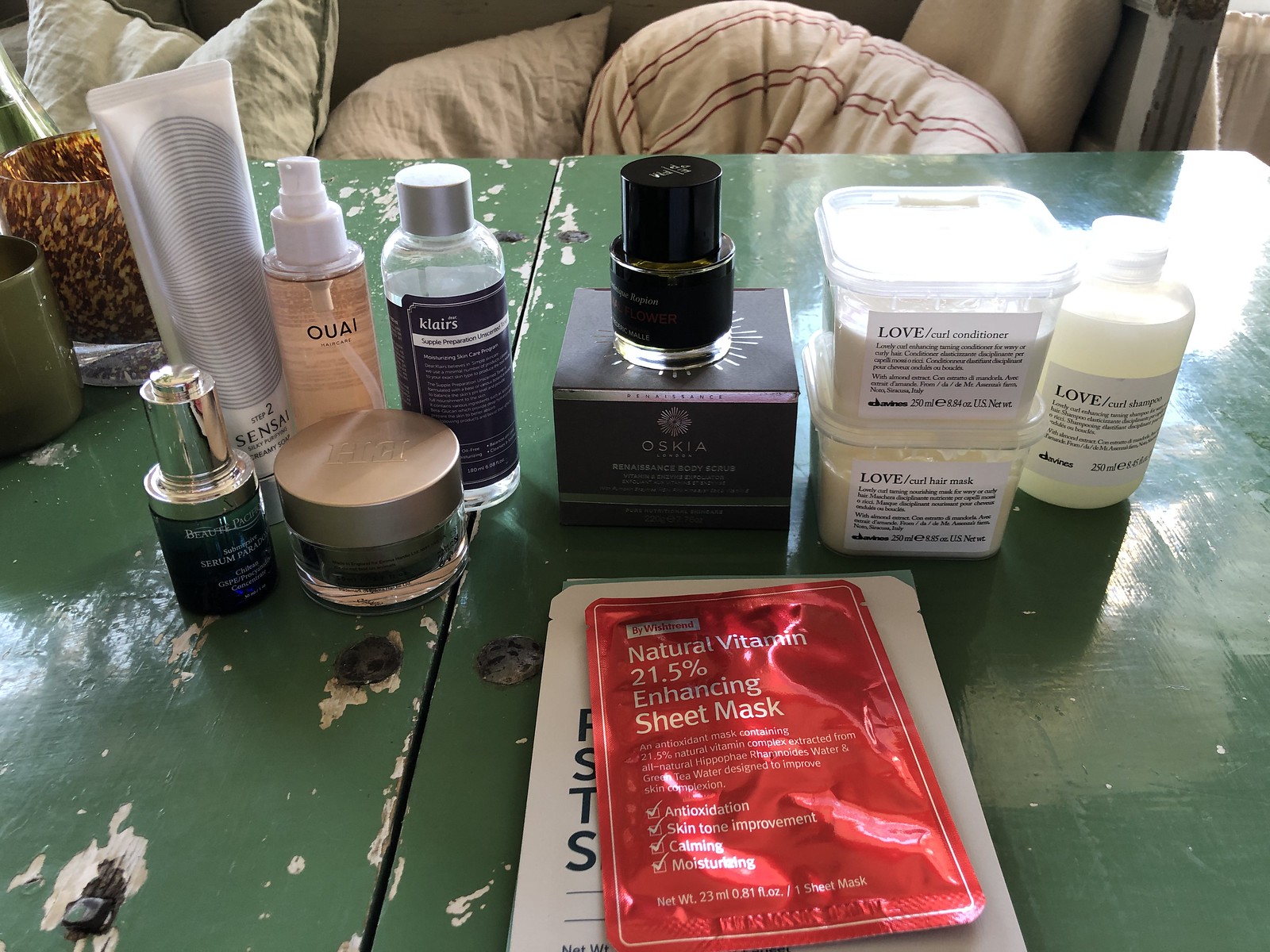On a roughly painted wooden table, adorned with flaking green-gray enamel and protruding nails, lies a diverse collection of beauty products. The background features soft, ivory-colored pillows, creating a contrast against the table’s rustic charm. 

Starting from the upper left corner of the table, a circular container sits with a possibility of holding a candle, accompanied by a green mug. Adjacent to these is a tube of lotion with the partially visible label starting with "S-E-N-S." Beside it, a spray bottle branded "Q-U-A-I" and a clear bottle with a silver lid labeled "K-L-A-I-R-S" filled with clear liquid, add to the variety of items. Below this grouping, a wider jar with a taupe screw-top cover is positioned next to a small bottle with a silver-toned top.

Prominently placed in the center is a square-shaped bottle with a black, two-tiered circular lid, displaying the brand "O-S-K-I-A" along with additional text beneath it. Flanking this centerpiece are two cube-shaped containers labeled "Love Curl Conditioner" and "Love Hair Mask," revealing white contents through their clear plastic exterior. Towards the right, another bottle with the "Love" label remains partially obscured. 

In the foreground, a white piece of paper with visible letters lies beneath a striking red packet that proclaims, "Natural Vitamin 21.5% Enhancing Sheet Mask," highlighting the curated collection on this quaint tabletop.